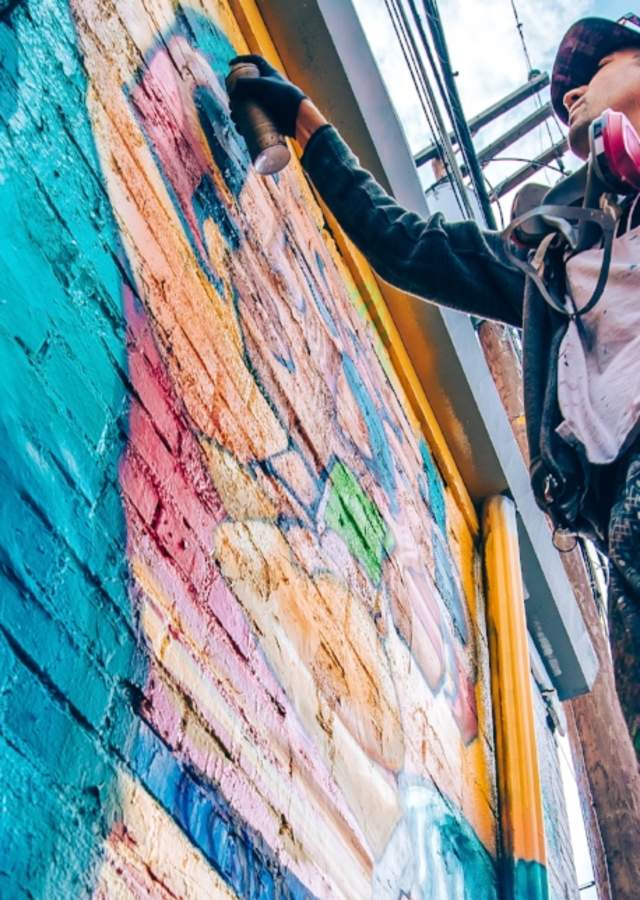In this striking image, we observe a male graffiti artist captured mid-action as he spray-paints a vibrant brick wall. The artist, dressed in a dark hoodie with a white shirt underneath, dark and white spotty pants, and a black cap with traces of pink spray paint, stands partially visible near the center-right of the composition. His protective respirator hangs loosely around his neck, indicating safety precautions. The wall, a rich canvas of diverse hues including blue, red, pink, yellow, orange, peach, and green, is covered in layers of intricate graffiti, creating a colorful mosaic. Particularly striking is the pink paint currently being sprayed from a can held close to the wall, complementing the myriad of other colors splashed across the bricks. A black glove on his hand suggests careful attention to detail as he works. The perspective of the shot, angled upwards, reveals his outstretched arm and the bottom of his chin and jawline, with a glimpse of blue sky and white clouds framing the scene from the upper right, adding an open, expansive feel to the urban artistry.